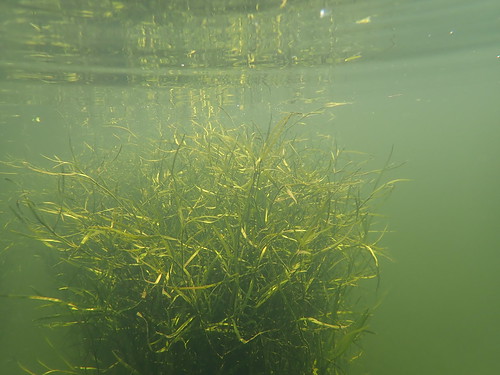Underwater photography reveals a dense, green mass of thin, vine-like plants or bush submerged in a lake or ocean, resembling long, tangled hair or spiny tendrils. The photograph, taken with an underwater camera, captures the plant’s thin stems and pointy leaves, with varying shades of green dominating the scene. The water is somewhat murky but clear enough to reveal the intricate details of the bush, which occupies the majority of the image, with the top section showing ripples and reflections on the water’s surface. Despite the slight cloudiness and blotchy appearance due to the underwater conditions, the sun’s rays penetrate through the water, adding an ethereal quality to the scene. The plant extends downwards into the shadows, with no other marine life or distinguishing features visible, creating a serene and isolated underwater landscape.